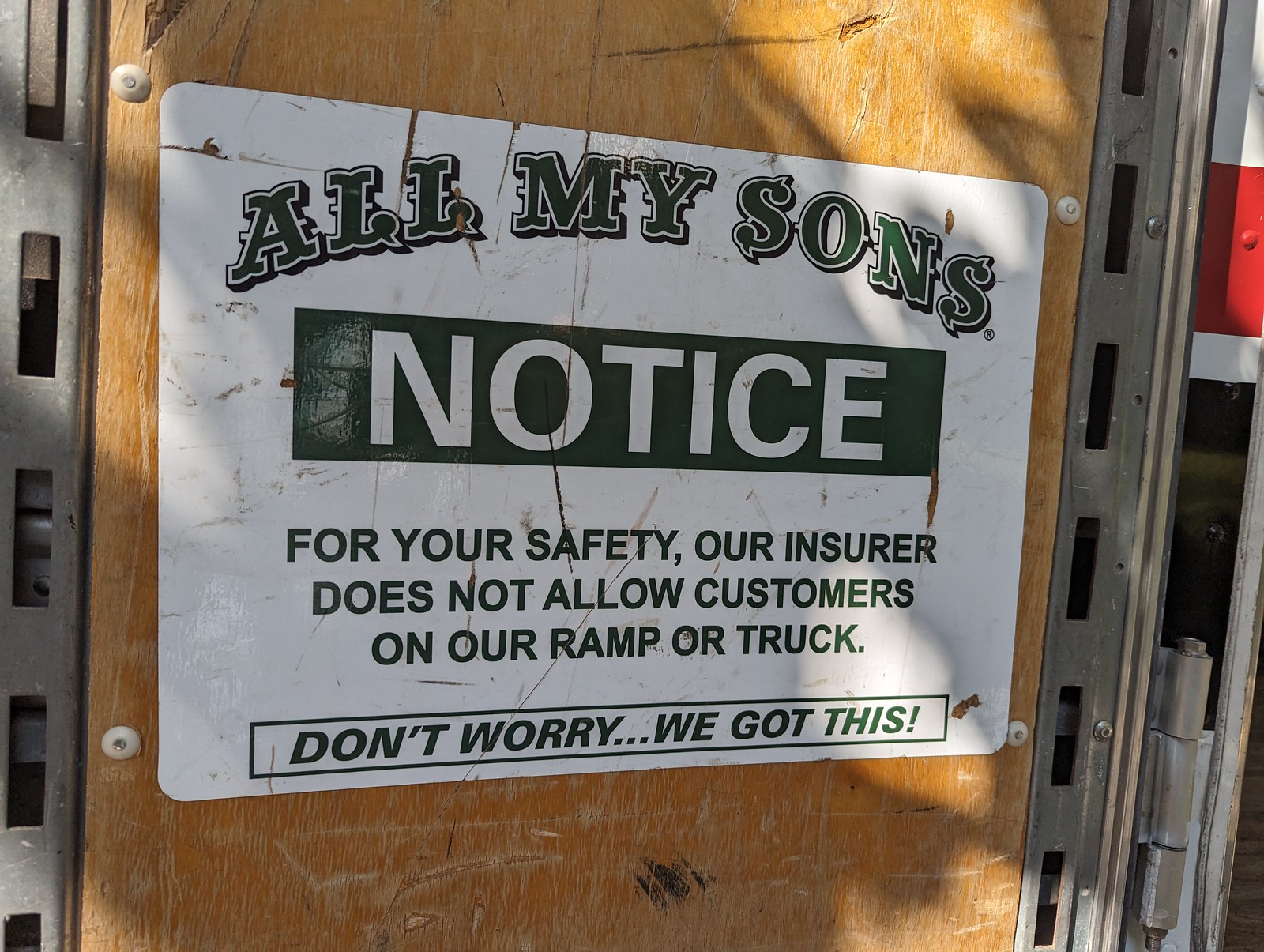The photograph features a weathered sign affixed to a rough, wooden structure with a metal frame, possibly a fence or the back door of a trailer. The sign, set against a brown board, has a white background and displays text in black and green. At the top, in italicized black text, it reads "Notice: All My Sons," denoting the name of the trucking company. Below this, a black horizontal banner highlights the word "Notice" in white text. Below the banner, in black text on the white background, the sign states, "For our safety, our insurer does not allow customers on our ramp or truck." At the bottom of the sign, enclosed within a rectangular outline, it reads, "Don't worry... we got this!" The overall message clearly warns against unauthorized access to the ramp or truck, ensuring safety protocols are followed. Although the sign appears worn and has been in place for a considerable time, its instructions remain clear.